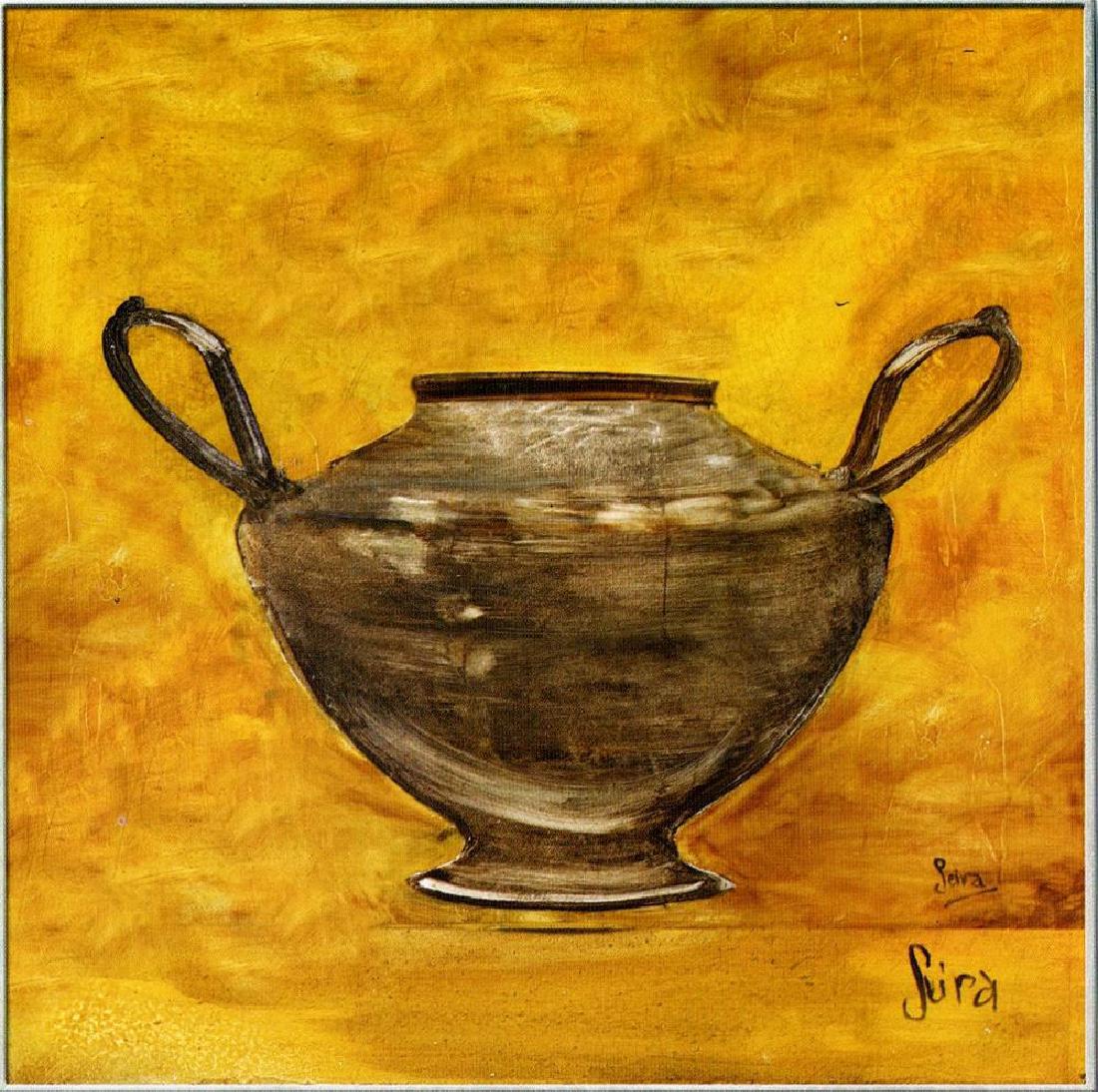The image depicts a painting of a metal vase that is primarily gold in color with dark brown painted accents. The vase is bowl-shaped with a small, round base, and it features two wing-shaped handles on each side. The opening of the vase matches the width of its base. The background of the painting consists of warm, golden hues mixed with brown and orange streaks, creating a dynamic, fiery appearance due to the visible brushstrokes. In the bottom right corner, the painter's signature, "Sura," is written twice: once in the upper area and once in the lower right area. The artist has used a streaky effect to render both the vase and the background, contributing to the lively feel of the artwork.